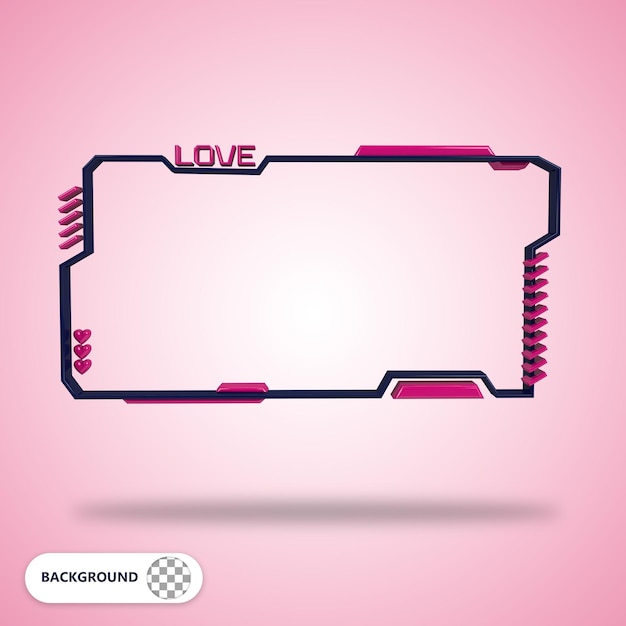This detailed, three-dimensional cartoon image features a visually intriguing scene. Dominating the foreground is a rectangular, black object that resembles a license plate. It is adorned with vibrant pink accents and prominently features the word "Love" in pink on the top left corner. Surrounding this central object are several floating hearts, adding an element of whimsy and affection.

The background of the image is a rich, solid pink, which gradually transitions to a whitish hue as it approaches the center, creating a subtle, glowing effect. At the bottom of the image, the word "Background" appears within a small circle designed like a chessboard, adding an interesting graphical element.

The rectangular shape appears to be suspended in mid-air, casting a soft, horizontal shadow on the ground below, which accentuates the three-dimensional aspect of the scene. Together, these elements combine to create a visually engaging and detail-rich composition that exudes a sense of warmth and love.